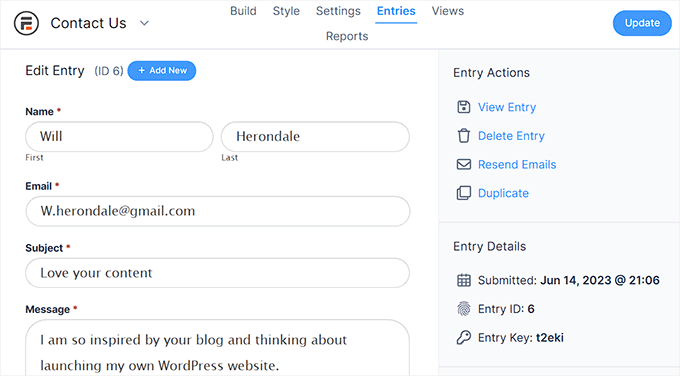The screen displays a form interface that is predominantly set against a white background. The right one-third of the screen is occupied by a vertical light blue box that contrasts with the white remainder. The entire screen is framed by a thin, pale light gray border.

In the top-left corner, "Contact Us" is prominently displayed in black text, accompanied by a drop-down arrow. To its left, there is an unbranded logo—a white circle outlined in black, featuring a black and orange design. Directly to the right of "Contact Us," various navigation options are presented in gray text: Build, Style, Settings, Entries, Views, and Reports. The "Entries" tab is currently selected, highlighted in bright blue with a corresponding underline.

On the far right of the header is a bright blue "Update" button with white text. Just below this header, a light gray line spans the width of the screen, providing a clear separation from the content below.

Below the navigation header on the left-hand side, "Edit Entry (ID6)" is displayed in black text. Adjacent to it on the right is a bright blue button that features a plus sign and the label "Add New" in white text. 

In the main form area, there are several input sections for user details:
- "Name" appears in black text with a red asterisk, indicating a required field. Below it are two text boxes labeled "First Name" and "Last Name," filled in with "Will" and "Herondale" respectively.
- The "Email" field also features a red asterisk and is filled with "w.herondale@gmail.com."
- The "Subject" field is marked as required and contains "Love Your Content."
- The "Message" field, similarly marked as required, contains the text, "I am so inspired by your blog and thinking about launching my own WordPress website."

To the far right, the light blue vertical box is labeled "Entry Actions" at the top in black text. Listed below in bright blue text are the actions: View Entry, Delete Entry, Recent Emails, and Duplicate.